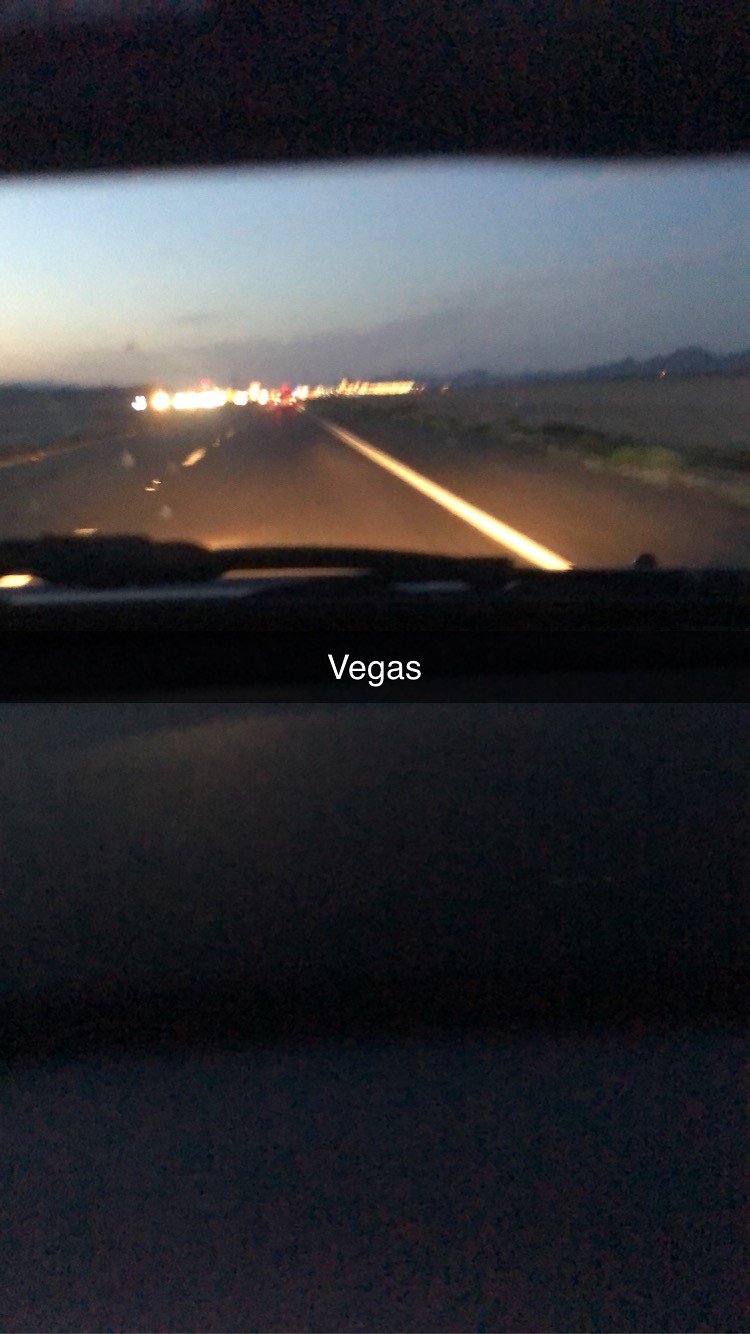This photograph, taken in a portrait orientation with a 16:9 aspect ratio, captures a scene from the back seat of an automobile, likely using a mobile phone. The bottom half of the image shows the vehicle's back seat, bathed in the dim light of either early dawn or dusk. The upper half reveals a view through the car's rear window, where a road stretches into the distance. The sky, adorned with faint clouds, creates a backdrop for a series of blurry lights, hinting at the hustle and bustle of a distant city. In the very center of the image, the word "Vegas" is prominently visible, suggesting the destination or theme of the journey. The overall ambiance of the photograph is dark and subdued, enhancing the mystique of the scene and the anticipation of the locale ahead.